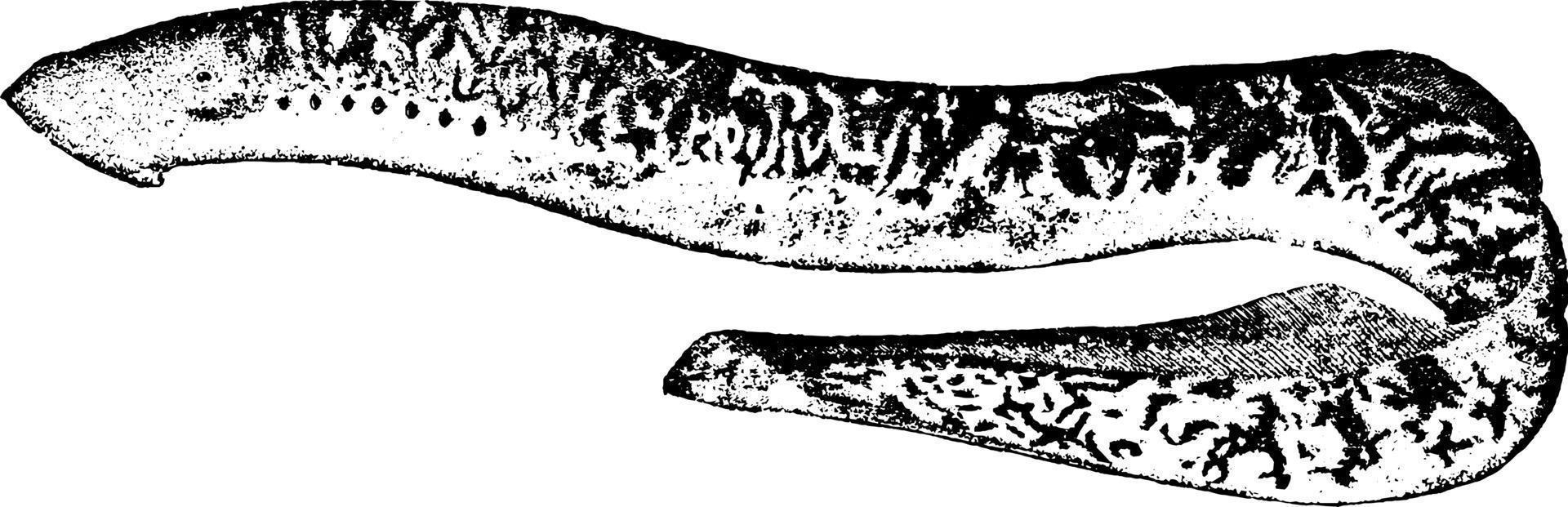The image depicts a black and white sketch of a long, slender creature, which appears to be a snake or eel-like animal with a somewhat curved body. Its entire form is detailed with white speckles or spots against a predominantly black body, and it has a white underbelly. The background of the sketch is completely white, highlighting the animal's distinct black and white patterns that resemble scales. The head of this creature is notably thinner or flatter than the rest of its body, with facial features such as eyes, mouth, or nose not clearly visible. It has no legs or appendages, and its elongated body pattern and structure suggest it could be a prehistoric creature or resemble large aquatic or serpentine animals like pythons or eels. The depiction captures intricate details like the scaled patterns and shading variations, enhancing its realistic yet enigmatic appearance.